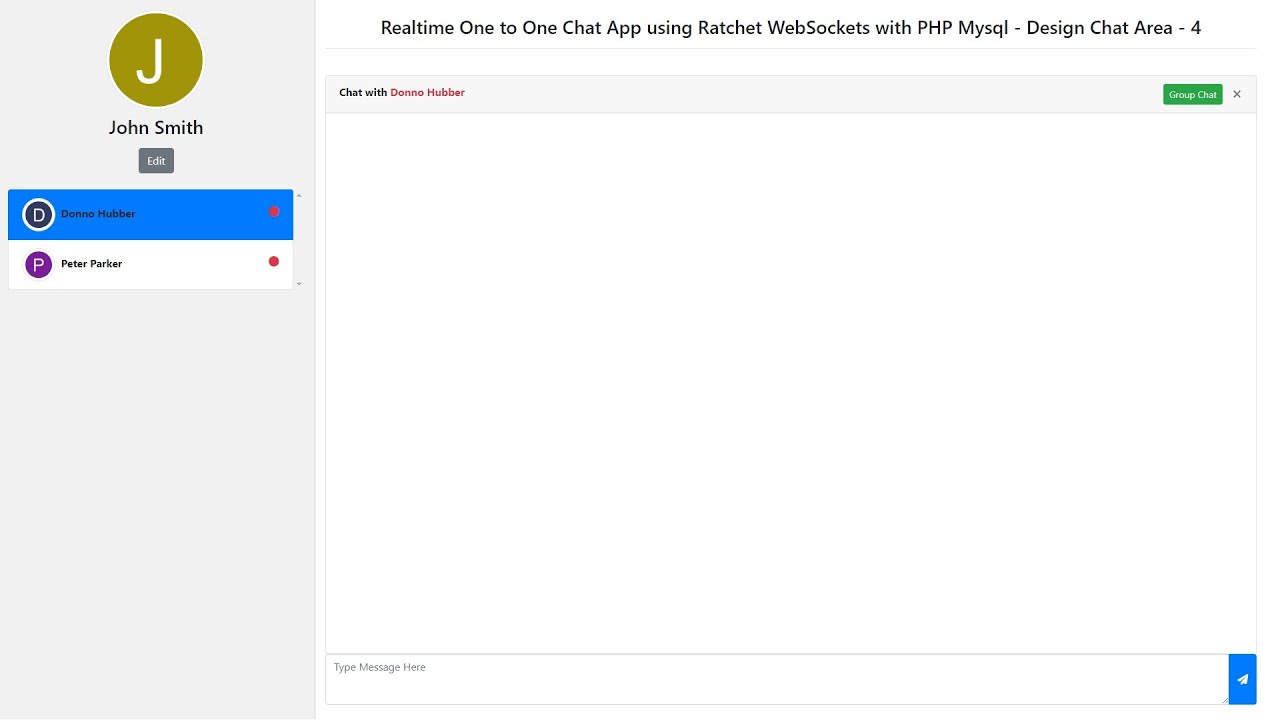In the image, Don Smith, Donna Hubber, and Peter Parker are participating in a real-time chat using a one-to-one messaging application built with Ratchet WebSockets and PHP. The chat interface, designed by Miskel, features a clean and intuitive layout. Donna Hubber is currently active in the chat area labeled "negative four," engaged in a conversation with Don. The interface prominently showcases chat input elements, including a message typing field and a send button. Bright red dots indicate the active status of users within the chat, creating a lively and engaging environment. The chat window has a distinct section titled "game chat X" where users can interact seamlessly.